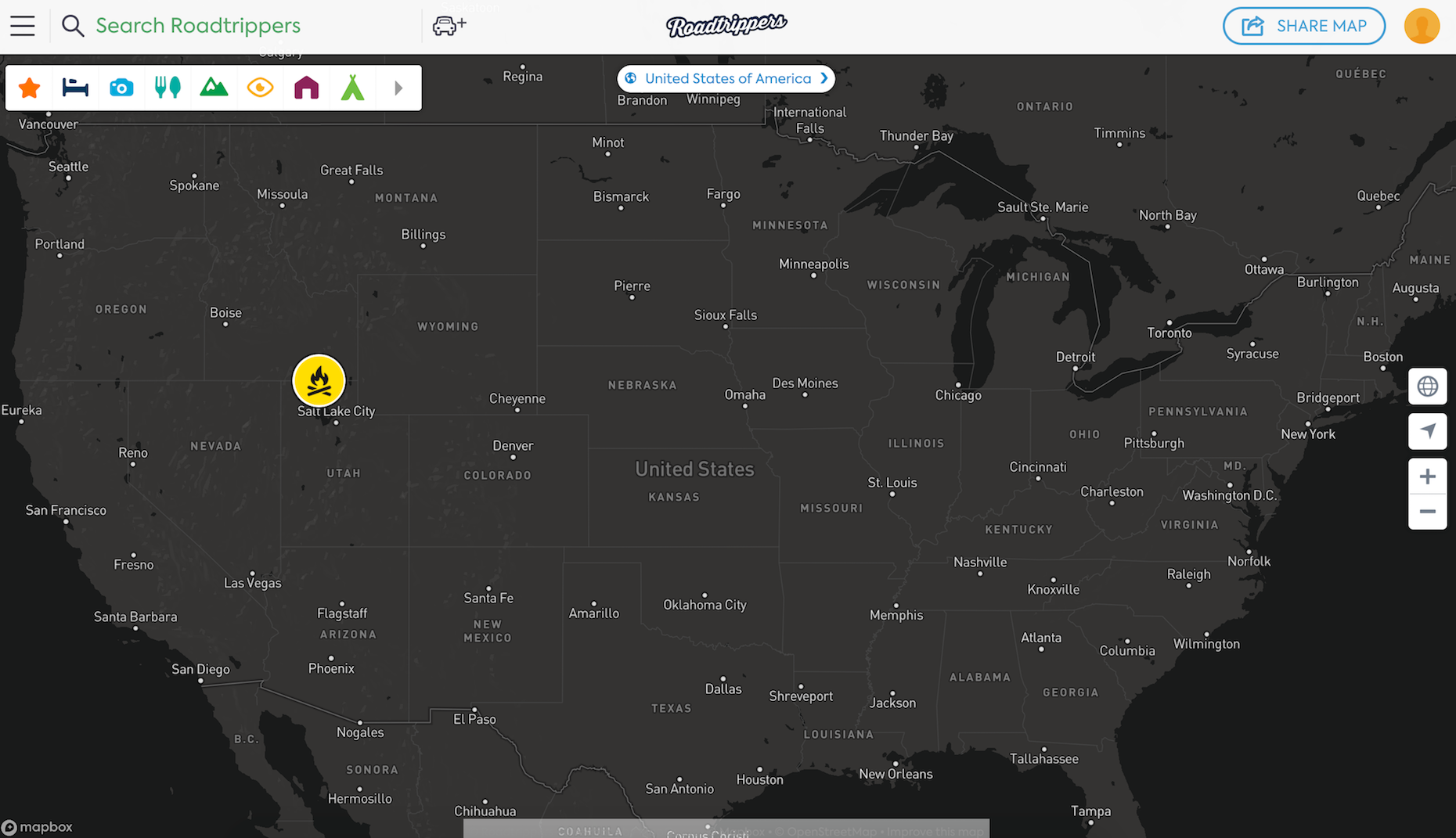A detailed screenshot of the "Roadtrippers" map interface is displayed. At the top of the screen, the menu bar is visible. In the upper left-hand corner, three parallel lines signify a menu option. To the right of this, there is a search field, followed by a small icon of a car with a plus sign next to it. Centrally located on the menu bar, the "Roadtrippers" logo is displayed. On the far right, there is a share map button, and next to it, an orange circle indicates a user profile.

Below the menu bar, the main display shows a map of the United States, highlighting various cities. Centered just under the menu bar, the label "United States of America" is evident. On the right side of the map, there is a vertical bar containing several icons: a star, a bed with a person in it, a camera, a fork and spoon, a mountain, a location services icon, a house, and a teepee or tent icon.

A specific point of interest is highlighted in Salt Lake City with a yellow circle featuring an icon that resembles a fire pit. This captivating screen provides a comprehensive overview and user-friendly interface for planning road trips across the United States.